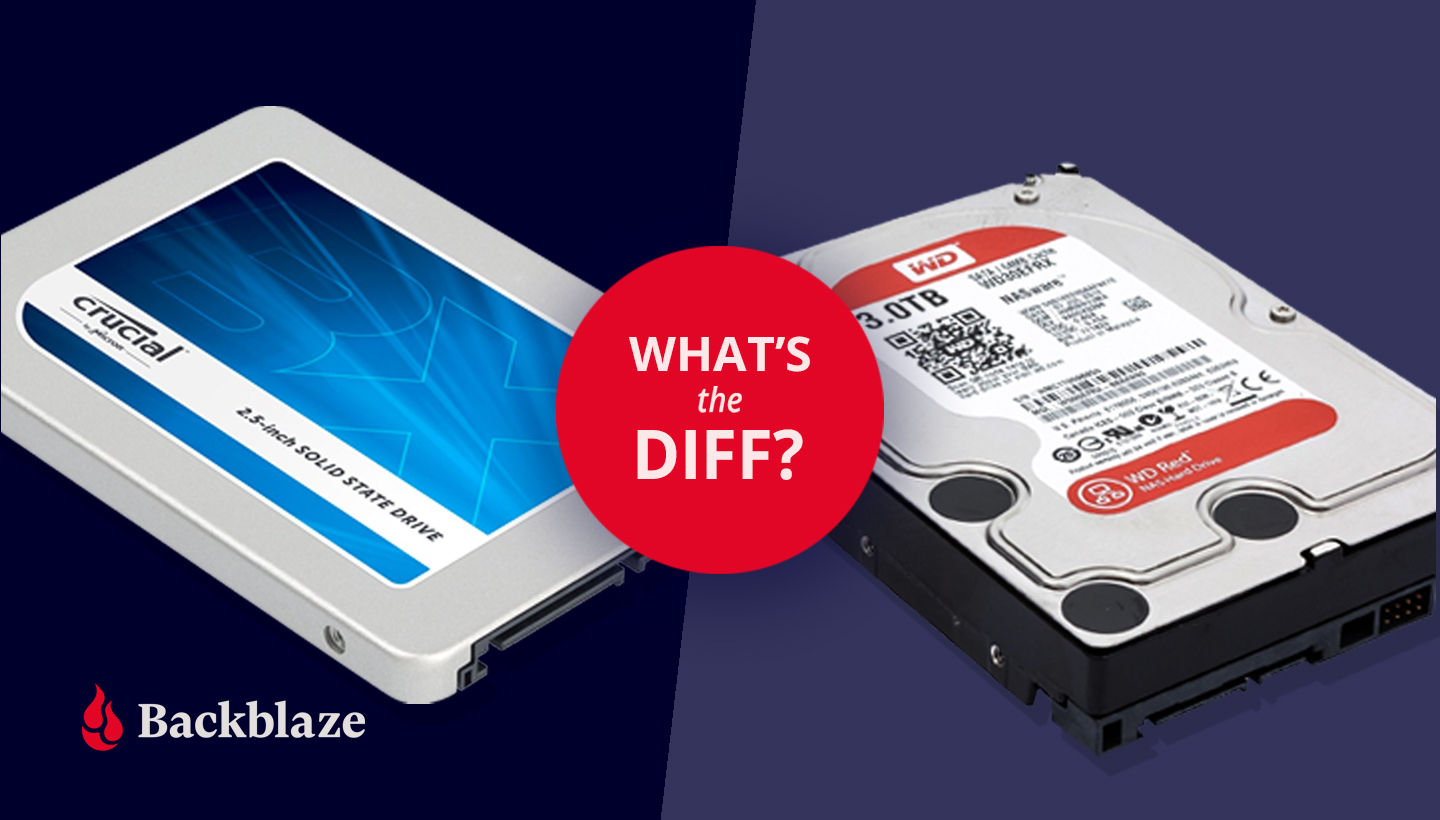This image, likely created by a digital publication such as an online blog or gadget magazine, is designed to compare two types of hard drives. The divided background features a dark purple hue on the left and a lighter purple on the right. Each half contains a different technological gadget: a Crucial branded 2.5-inch solid-state drive (SSD) on the left, and a Western Digital 3.5-inch platter-based hard drive (HDD) on the right. Both devices are silver in color, with the SSD showcasing predominantly blue labeling and the HDD featuring a white label with red and blue accents, plus various fine print elements including barcodes and a QR code. Central to the image is a red circle with white text that reads "What's the diff?", likely signifying a comparison between the two hard drives. This phrase stands for "What's the difference?" At the bottom left corner, the logo for Backblaze appears, featuring a red flame symbol and white text, indicating that Backblaze may be either the publication or retailer of these products. This editorial graphic is probably used as a header for an article that contrasts the performance and features of SSDs and HDDs.